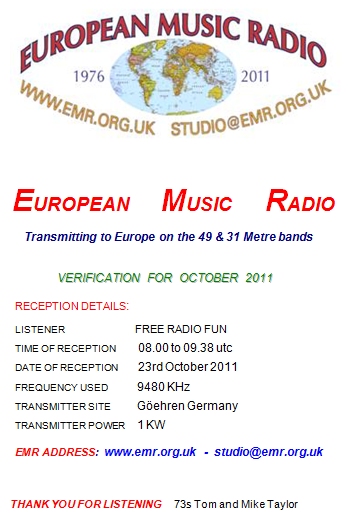This is an advertisement poster for European Music Radio, featuring the timeframe 1976 to 2011 prominently displayed alongside a central globe illustration. The website (www.emr.org.uk) and email address (studio@emr.org.uk) are clearly listed above and below the globe. A bold red header states "European Music Radio," and a blue line below it declares "Transmitting to Europe on the 49 and 31 meter bands." The poster also highlights verification details for October 2011 in green font, followed by reception specifics including the listener's data, date and time of reception, frequency used, transmitter site, and power in black text. Notably, it mentions the free fun radio event held on October 23, 2011, from 08:29 to 09:38 UTC on 9480 kHz, transmitted from Goren, Germany with a power of 1kW.